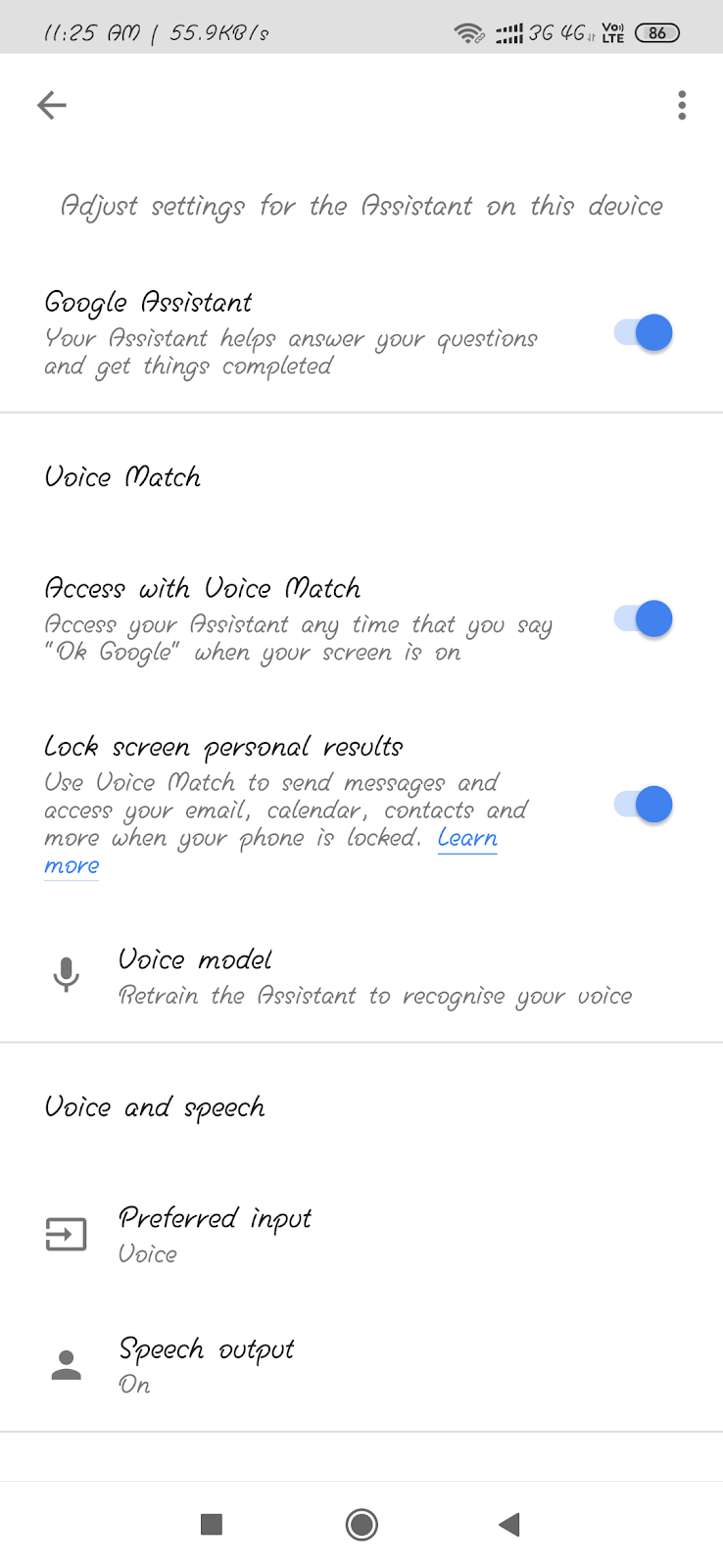The image showcases an Android phone with a custom interface featuring a hand-drawn, cursive-like font in black text. The device's information bar at the top is on a gray background, showing the time (11:25 a.m.), battery icon, and multiple connectivity indicators including LTE, 3G, 4G, and Wi-Fi. The data speed displayed is 55.9 kilobytes per second.

Below this, the main screen of the phone's settings application is visible against a white background. The heading reads, "Adjust settings for the assistant on this device," indicating the section pertains to Google Assistant settings. Three options are shown with blue toggles, activated to indicate they are turned on: "Google Assistant," "Access with Voice Match," and "Lock screen with personal results." 

Further down, the section "Voice Model" suggests users can retrain the assistant to their voice, accompanied by a microphone icon. Another section named "Voice and Speech" highlights settings for preferred input, both set to "voice" and "speech input," all switched on.

At the bottom of the screen, the navigation bar is evident, featuring the familiar Android icons: a back arrow, a home circle, and a recent apps square, all in dark gray against a white background. This affirms the device is running an Android operating system.